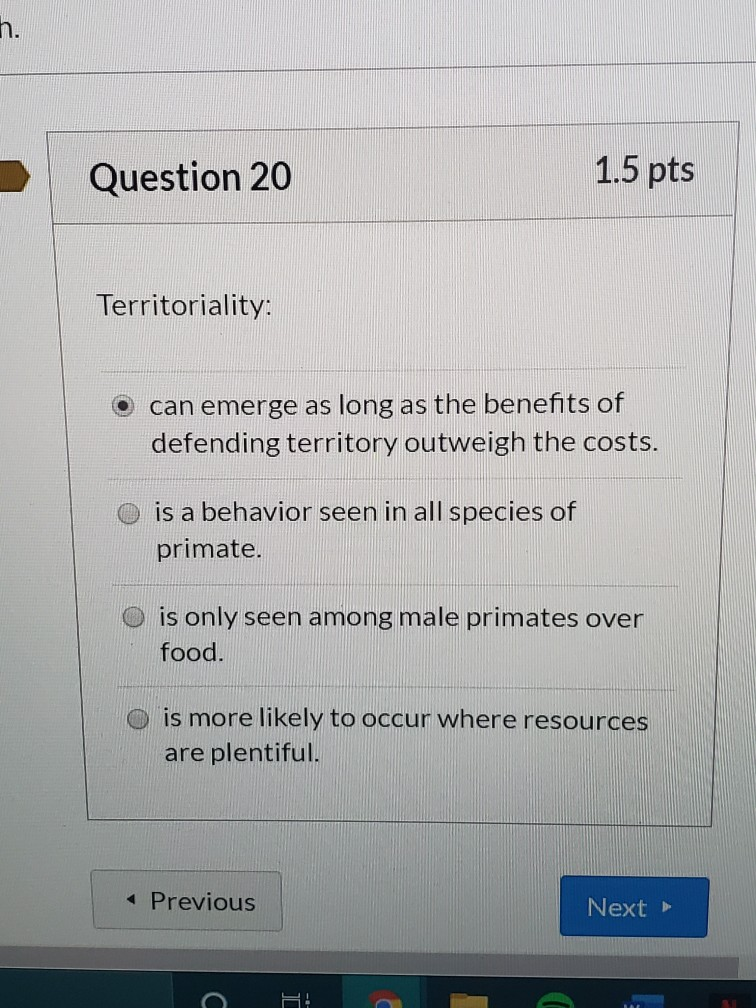The image displays a computer screen featuring a website with a predominantly white background. In the top left corner, there is an icon that appears to be an incomplete letter 'N' or 'H,' partially obscured, followed by a period. Below this icon, there is a horizontal line leading to a thick, filled-in arrow colored brown, pointing to a rectangular section.

The rectangular section is part of a quiz or assessment interface. The top banner of this section showcases the text "Question 20, 1.5 PTS" in bold, with "Question 20" on the left and "1.5 PTS" on the right.

Underneath the banner, the screen displays the term "Territoriality" in bold, followed by a colon. Below this term, four multiple-choice definitions are presented:

1. "Can emerge as long as the benefits of defending territory outweigh the costs."
2. "Is a behavior seen in all species of primate."
3. "Is only seen among male primates over food."
4. "Is more likely to occur when resources are plentiful."

The first option is marked as selected, indicated by a filled-in circle next to its text.

At the bottom of the question section, there is a navigation bar with the option "Previous" on the left and "Next" on the right. The "Next" option is highlighted with a blue background and features an arrow pointing to the right.